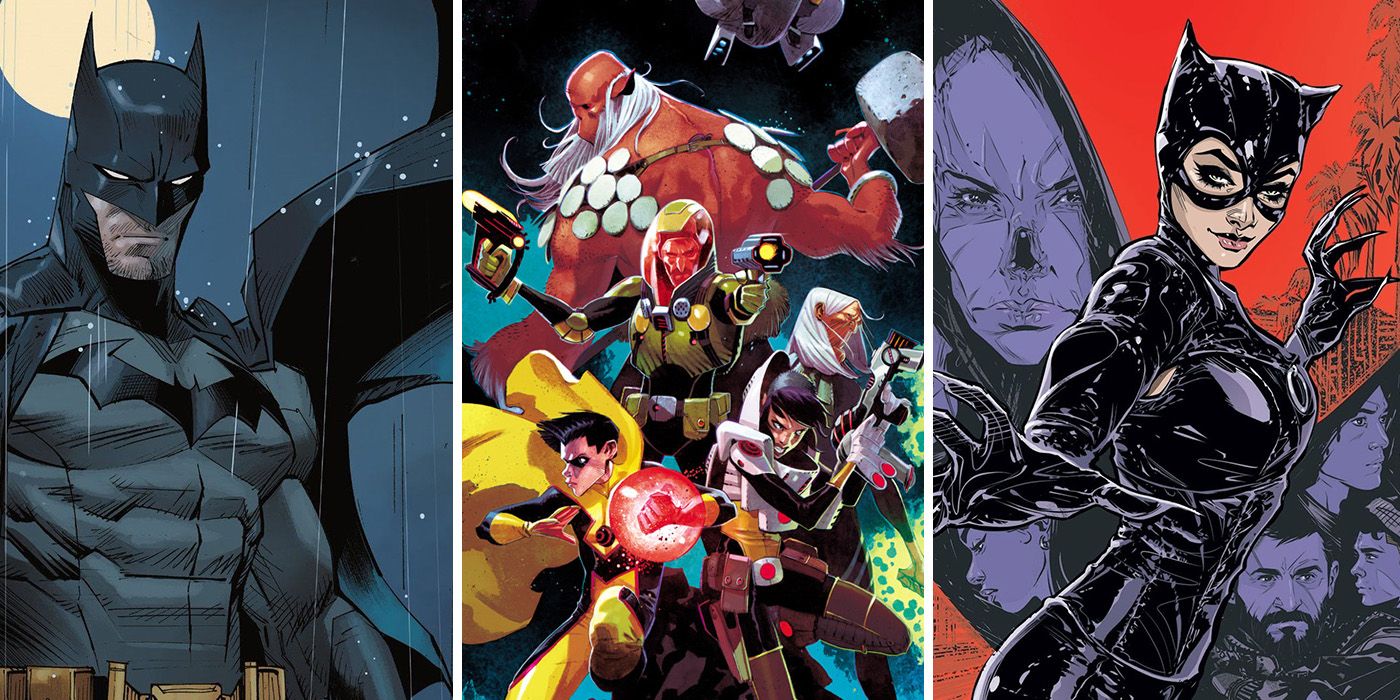This landscape-oriented image is divided into three distinct comic book-style panels by white lines. The left panel depicts Batman in his classic gray armor outfit with a flowing cape and a gold belt, standing solemnly with his head slightly bowed. The night sky behind him is dotted with stars, and rain pours down, adding to the somber mood. The moon glows brightly above his head.

In the middle panel, five superheroes stand together, each in dynamic poses. Among them is a character with a yellow cape, another with red skin and decorative shoulder pieces, a figure with silver hair who exudes a sense of power, and a space-themed character with green elements in their costume. An individual with a large hammer reminiscent of Thor's Mjolnir is also notable, adding to the eclectic group.

The right panel features Catwoman in a striking, tight black leathery outfit, complete with her iconic mask, accentuating her feline allure. Her arms are extended, one behind her and one in front, showcasing her clawed gloves. The background is split, with a red upper section containing silhouettes of characters tinted in blue. There are also palm trees and buildings faintly visible, adding depth to the backdrop.